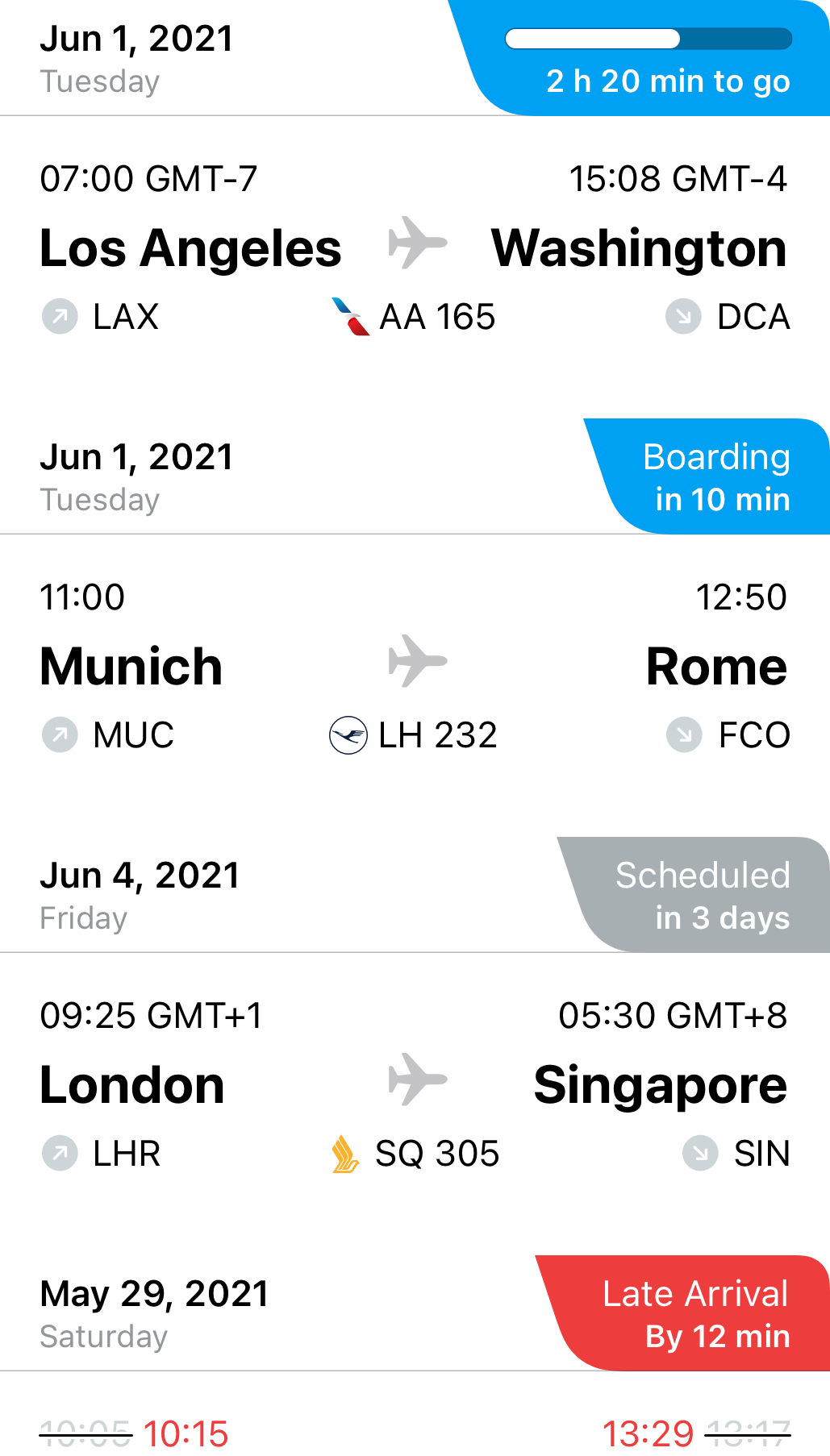The image displays a detailed digital screen layout, segmented into multiple sections arranged vertically. At the top left, the screen shows the date "June 1st, 2021, Tuesday." To the top right, there is a prominent white slider. Just below, the text "2H, 20 minutes to go" indicates the remaining time to an event.

Moving down to the next section, on the left, the time "07:00 GMT-7" is displayed, and on the right, "15:08 GMT-4." Below these times, the screen labels the location "Los Angeles" with a gray airplane icon to its right, followed by the destination "Washington."

Further down, the screen reads "LAX" in the left-middle section, "AA-165" centered, and "DCA" to the right. Underneath "AA-165," the date "June 1st, 2021, Tuesday" repeats, with the right side indicating "boarding in 10 minutes." At the very bottom, the time "11:00" is displayed, finalizing the information presented on the screen.